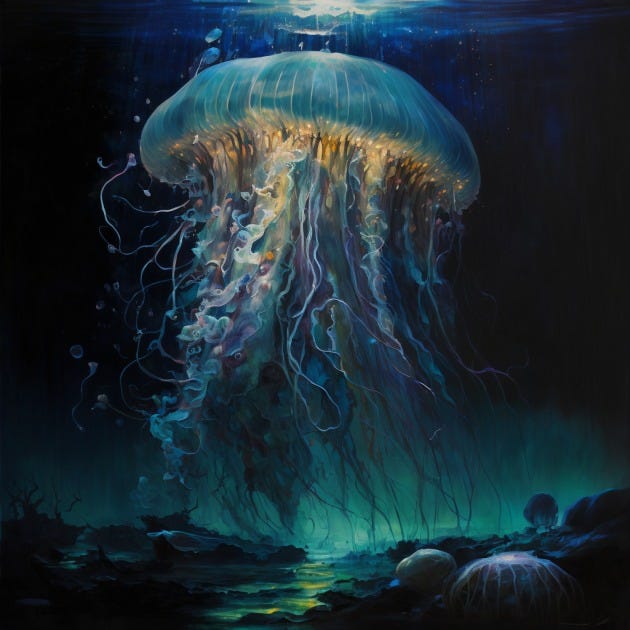The image is a highly detailed digital painting of an immense jellyfish, nearly spanning the entire height of the canvas as it appears to reach from near the ocean floor to just below the water’s surface. Set in the dark, deep blue waters with a rich interplay of shadows and light, the jellyfish is a striking centerpiece. The smooth, mushroom-like cap of the jellyfish glows with a bioluminescent teal, accented by gold and white highlights beneath it. 

The jellyfish's hundreds of tentacles unfurl gracefully, displaying a captivating array of colors including blue, yellow, white, purple, pink, and teal. These tentacles flow downward with a liquid-like smoothness, adding a dynamic motion to the still image. 

Above the jellyfish, a luminous "R" shape of light appears, perhaps refracted moonlight, adding to the ethereal quality of the scene. The jellyfish itself emits a bright glow from its center, projecting light both upwards and downwards, creating a blue and greenish near-transparent illumination that enhances the painting's depth and mystery.

At the bottom right of the image, indistinct elements resembling rocks or potentially other sea creatures add texture to what seems to be the ocean floor, shrouded in the dim glow from the jellyfish. Scattered bubbles and a faint scattering of illuminated particles contribute to the intricate, almost otherworldly ambiance of this deep-sea tableau.